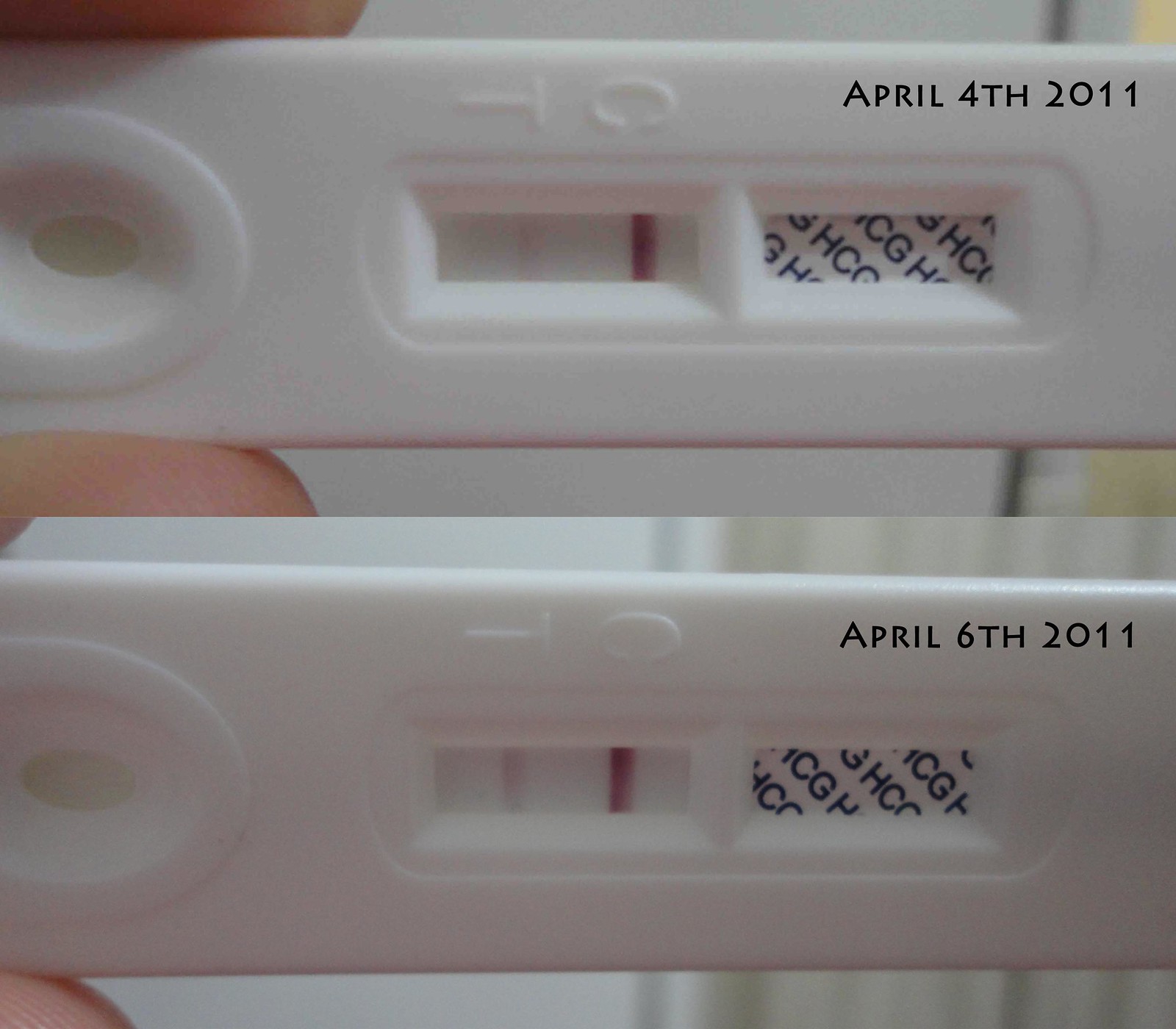This image features two nearly identical photographs, each showing a rectangular, plastic medical testing device, likely a home pregnancy test. The device has a circular window on its left side that appears clear in both images. Centrally located on the device are two rectangular windows. In the top photograph, a red bar is prominently visible beside a letter "C," while a faint red bar is discernible next to the letter "T." The label "HCG" is printed to the right of these windows, indicating the test's function related to human chorionic gonadotropin hormone detection. Both images display the same red bars in the rectangular windows. The only discernible difference between the images is the date stamp: the top image is dated April 4th, 2011, and the bottom image is dated April 6th, 2011. Despite the differing dates, the test results appear consistent across both images.